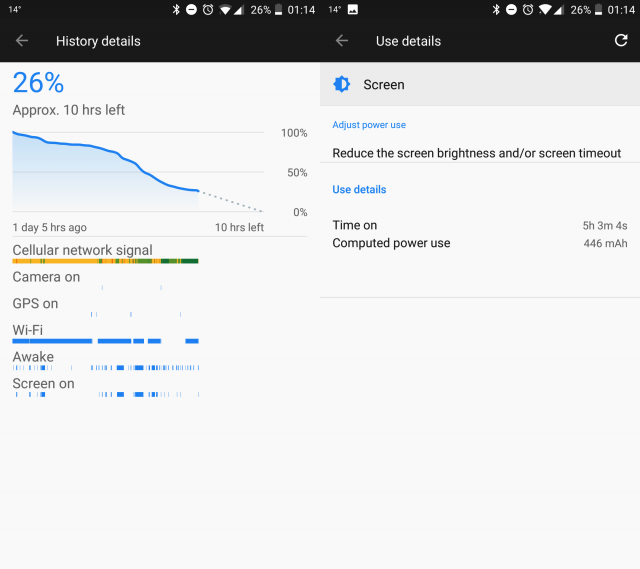The image depicts the settings section of a phone application, focusing on the "History Details" tab. Central to the display is a graphical representation of battery usage, illustrating that the device currently has 26% battery remaining, equating to approximately 10 hours of usage left. The graph charts a steady decline from 100% to 0%, with a dotted line marking the trajectory once the battery falls below 50%. Annotations indicate that 1 day and 5 hours have passed since the last full charge, and 5 hours of battery life remain on the left side of the graph.

Further details beneath the graph provide insights into specific energy-consuming activities. The list includes categories such as cellular network signal, camera on, GPS on, WiFi awake, and screen on. Additional options for managing battery life, such as reducing screen brightness and screen timeout durations, are listed below.

Finally, the "Usage Details" section quantifies the time on battery as 5 hours, 8 minutes, and 4 seconds, with computed power consumption measured at 446 mAh.